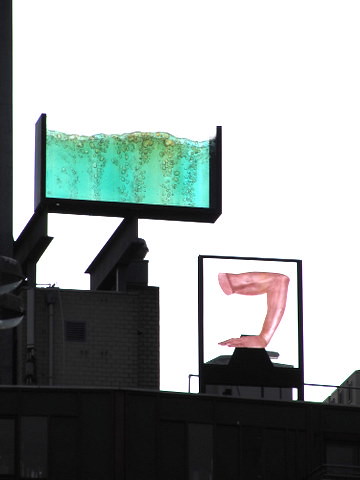The image depicts an abstract, digitally created scene set against a stark white, empty background. Dominating the lower portion is a dark, almost black structure that extends horizontally across the frame, suggestive of a wall or the roof of a building. On the right side of this structure, an arm emerges and bends at the elbow, with the hand extending downward as though pressing a button on the roof's surface. To the left, another part of the dark building structure rises up and features two unique elements: one, a rectangular black-framed open-top container that holds a sheet of bubbling water, and two, more ambiguous architectural forms that intersect and balance, contributing to the overall surreal atmosphere. The contrast between the black elements and the white void enhances the interpretive nature of the artwork, inviting viewers to explore its minimalist yet compelling visual narrative.